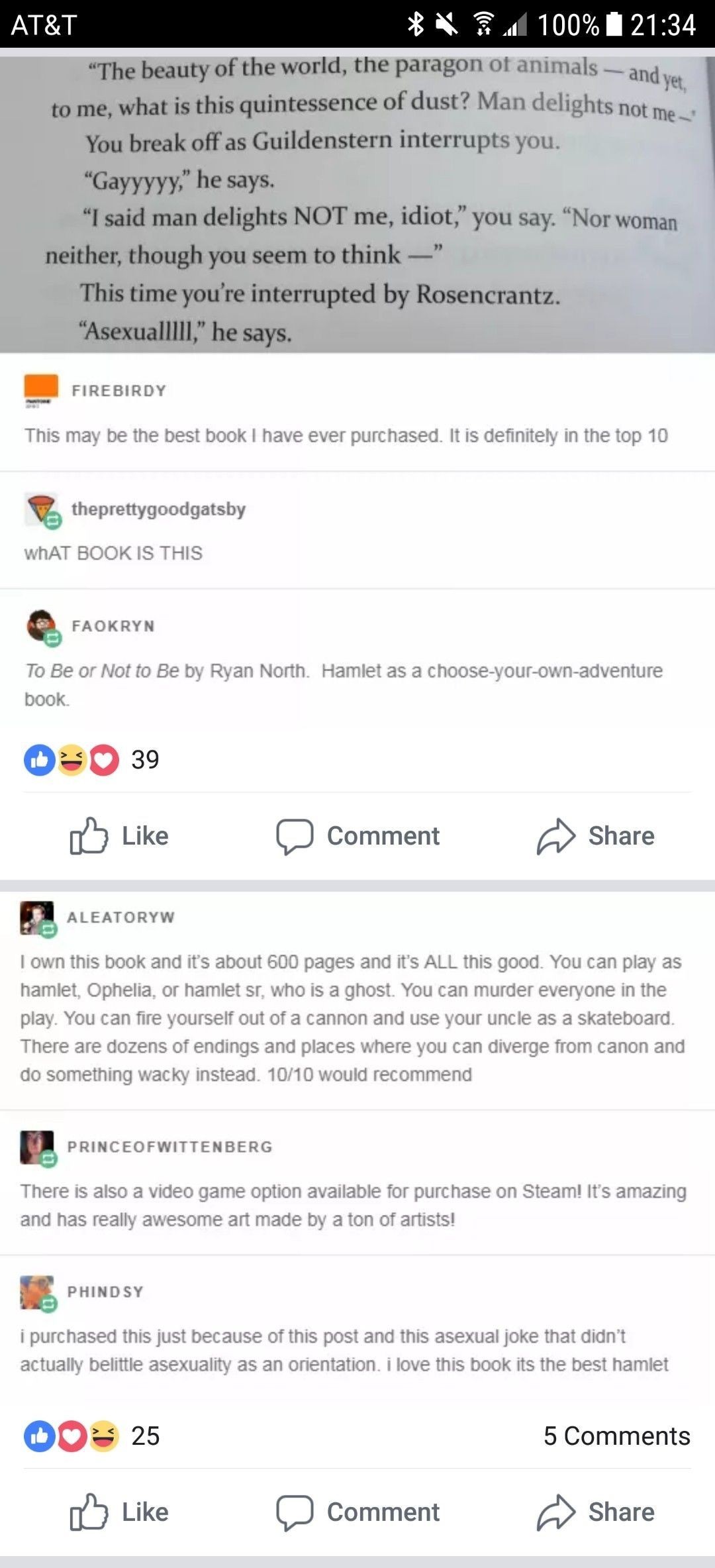A screenshot from a cell phone captures a web page featuring a lively chat conversation between several users. The phone toolbar at the top of the image indicates an AT&T connection, with a full battery at 100% and the time displayed as 9:34 PM (2134). Below the toolbar, a gray box contains text quoting a modified passage from Shakespeare’s "Hamlet," showcasing a humorous exchange involving characters Gildenstern and Rosencrantz.

Following the quote, the chat transitions into a discussion on the website FireBirdie. One user enthusiastically comments, "This may be the best book I have ever purchased. It is clearly in the top 10." Another user, "the pretty goody gaspy," inquires, "What book is this?" to which "Fayor Crenn" responds, "To Be or Not to Be by Ryan North, Hamlet as a choose-your-own-adventure book." The conversation humorously suggests a modern, possibly LGBTQ+ inclusive adaptation of Hamlet, reflecting a blend of classical literature with contemporary, interactive storytelling.